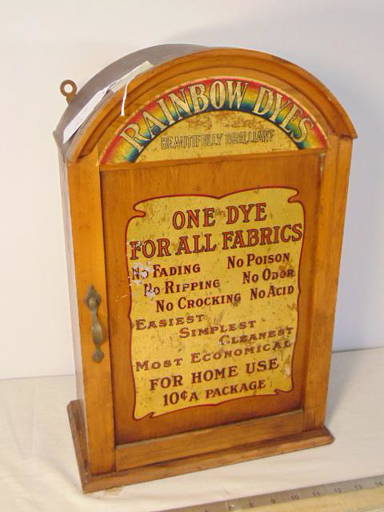This photograph features a small, antique wooden cabinet with a distinct rounded top, resembling the shape of a jukebox. The cabinet, aged and yellowish in color, has a front door adorned with a handle on the left side for opening. At the top of the cabinet, in faded arching print, the words "Rainbow Dyes" are written in white with a rainbow behind them. Below this, the front door boasts a detailed, multi-colored print within a yellow-bordered section that reads: "One dye for all fabrics. No fading, no ripping, no crocking, no poison, no odor, no acid. Easiest, simplest, cleanest, most economical for home use. 10 cents a package." This text is presented in a mix of red and black colors, giving it a vibrant yet antique look. The cabinet likely served as a dispenser for fabric dye packets, costing ten cents each, and was designed for practical home use, emphasizing its no-nonsense, user-friendly features.